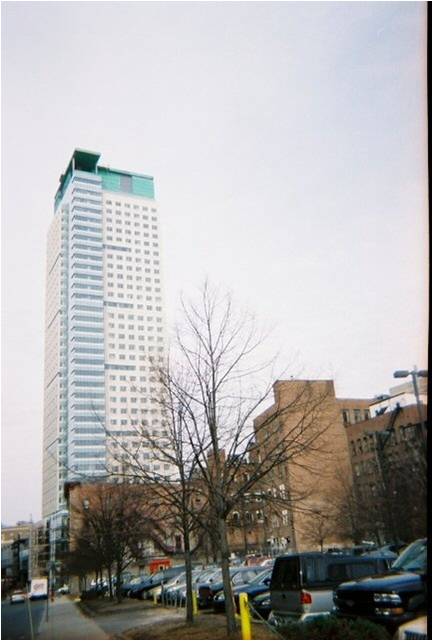The photograph captures a winter urban scene dominated by a tall, white skyscraper with green-tinted glass near the top, towering over several shorter, interconnected, light brown brick buildings. The skyscraper, possibly a hotel, showcases rows of rectangular windows and features a distinctive grey section with longer horizontal windows on its side. The mundane, gray sky adds to the wintry ambiance, while the leafless trees in the foreground further emphasize the season. Below, a paved parking lot is filled with cars reminiscent of the 1990s or 2000s era. Yellow parking bolsters line the area to prevent cars from encroaching onto the adjacent sidewalk, which runs along the bottom left of the image, separating the parking lot from a city street where a bus and a car traverse in the distant background.